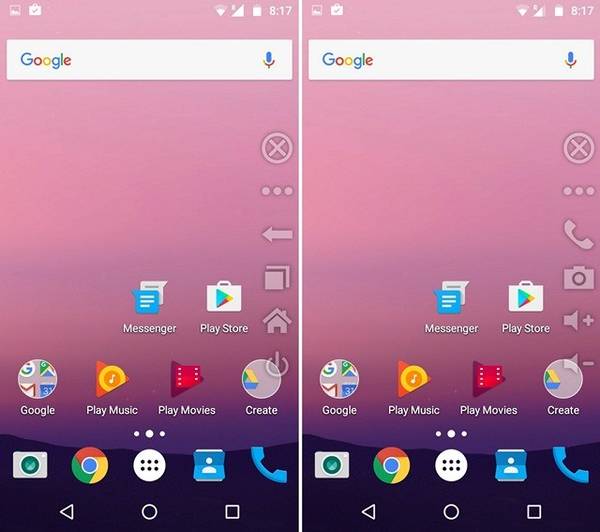The image consists of two side-by-side screenshots arranged in two columns, displaying nearly identical smartphone home screens with subtle differences. Both screenshots feature a pink background gradient transitioning to dark purple. In the upper right corner of each screenshot, there is a time stamp reading "8:17," indicating the screenshots were taken in quick succession.

Across the top of both screenshots, there is a Google search bar with a Google icon on the left and a microphone icon on the right. Below the search bar, the next row shows an "X" icon enclosed in a circle.

The row beneath contains three dots, but the content varies between the two columns. In the left screenshot, this row has a back arrow icon, while the right screenshot replaces this with a phone icon. Directly below these, the left column features an icon of two overlapping pieces of paper, whereas the right column substitutes this with a camera icon.

In the third row, both columns display Messenger and Play Store icons; however, the left column ends the row with a house icon, while the right column has a plus symbol for volume control. Underneath these icons, the left column has an icon that appears to represent location, while the right column shows a minus symbol for volume control.

The remainder of both screenshots displays typical phone app icons, with no further variations between the two columns.